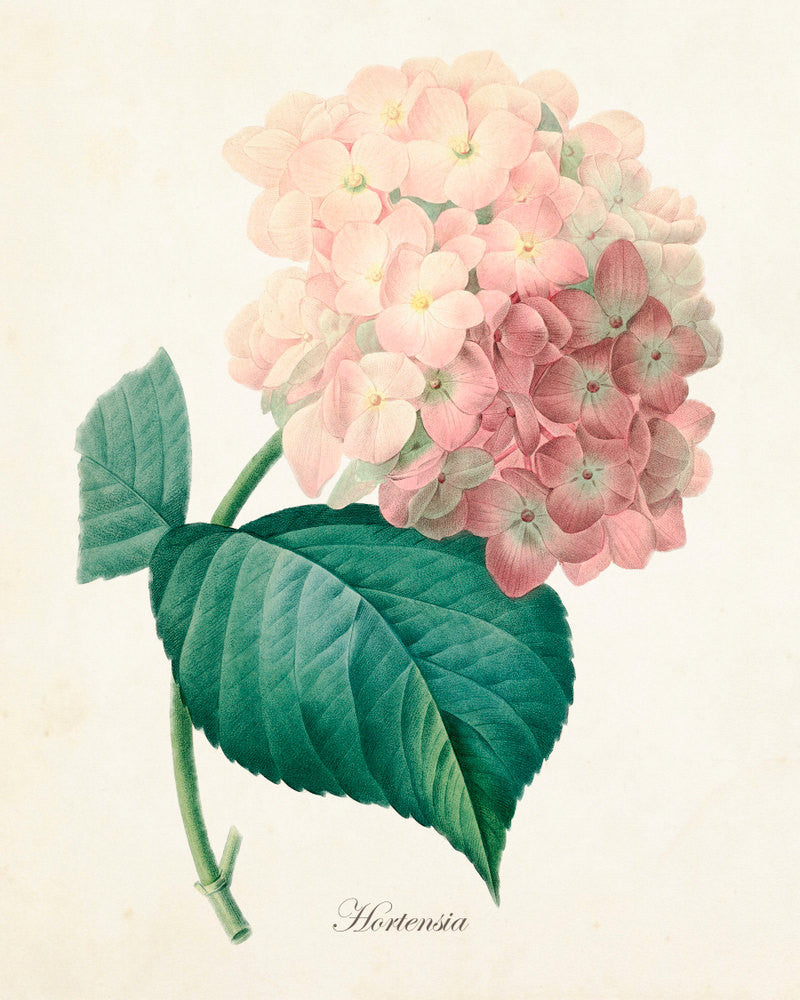This illustration, executed with meticulous detail on light pink or beige cardstock, depicts a single stem of a pink hydrangea, labeled "Hortensia" in black cursive at the bottom. The hydrangea blossom, composed of numerous tiny flowers with yellow centers, forms a circular bouquet on the stem. The petals transition from light pink at the top to darker pink at the bottom, accentuating its realistic appearance. Flanking the stem are two large, dark green, heart-shaped leaves with scalloped edges, creating a vivid contrast against the delicate petals. The end of the stem is cut off in the image, and the overall impression is one of scientific precision, suggesting this illustration might serve as a reference for botanists.